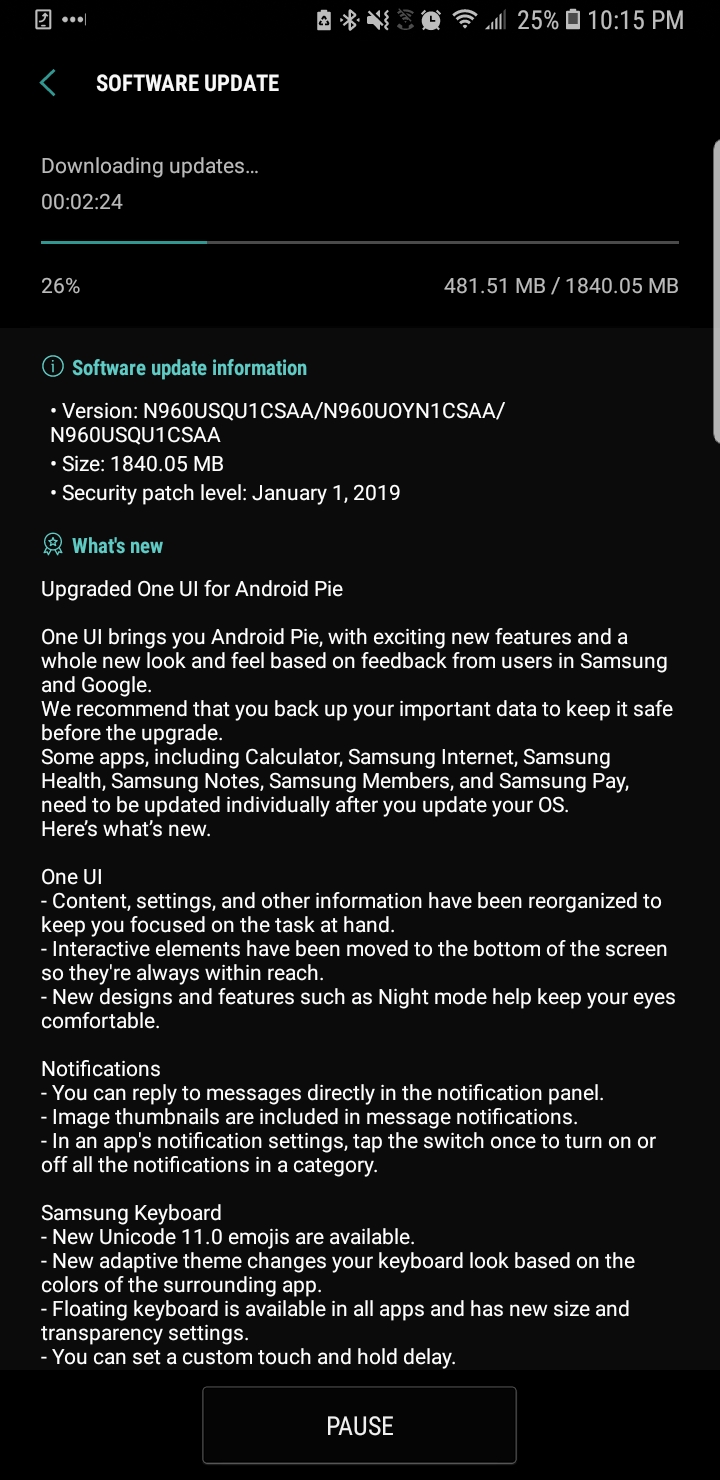**Screenshot of an Android Phone Software Update**

The screenshot displays an Android phone with a predominantly black background. At the top is a left arrow icon followed by the text “Software Update.” Beneath this, the words “Download and Install” are shown, indicating that a software update is in progress. A message reads “2 minutes 24 seconds remaining,” accompanied by a progress bar currently filled to 26%, with the data transfer rate highlighted as “481.51 MB / 1840.05 MB.”

Below the progress bar, there is an information symbol next to the text “Software Update Information.” Detailed update version numbers are listed as “N960USQU1CSAA / N960UOYN1CSAA / N960USQU1CSAA.” Further down is an award symbol, and the section titled “What’s New” outlines the upgraded features of One UI for Android Pie.

The description specifies that One UI introduces Android Pie with various new features and a revamped look and feel based on user feedback from Samsung and Google. Users are advised to back up their important data before proceeding with the upgrade.

Highlighted apps that need to be updated individually post OS update include Calculator, Samsung Internet, Samsung Health, Samsung Notes, Samsung Members, and Samsung Pay.

Key new features listed are:

- **One UI**: Enhanced organization of contacts, settings, and other information to maintain user focus. Interactive elements are repositioned to the bottom of the screen for easier access. New designs and features, such as Night Mode, are introduced to reduce eye strain.
- **Notifications**: Users can now reply to messages directly from the notification panel, which includes image thumbnails. The apps' notification center allows toggling notifications on or off for different categories with a single switch.
- **Samsung Keyboard**: Introduction of Unicode 11.0 emojis. The adaptive theme adjusts the keyboard color based on the surrounding app. The floating keyboard is available in all apps with new customization options for size and transparency. Users can set a custom delay for touch and hold actions.

At the bottom of the screenshot is a black button labeled "Pause," allowing the user to halt the update process if needed.